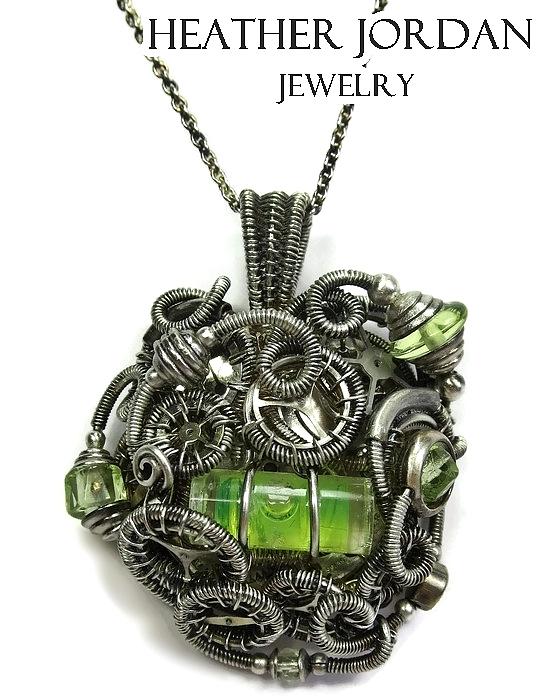This detailed, color photograph showcases an advertisement for Heather Jordan Jewelry. The image features a stunningly intricate silver necklace against a white background. The fine silver chain, visible from both the upper left and upper right corners, elegantly loops around a complex pendant. The pendant is a masterpiece of design, composed of numerous silver metal coils in varying circular shapes, and corrugated tubes intricately wrapped around each other. At its center, encased within the coils, lies a clear cylindrical container. Inside this transparent core is a green element resembling the bubble level used in construction, complete with vertical lines and a small air bubble. This central green indicator is flanked by additional green ornamental pieces shaped like triangles or small bells, adding a touch of color and creativity to the overall design. The pendant's sophisticated structure is perfectly highlighted by the minimalistic white background. At the top of the image, in bold, black, all-capital letters, the text "HEATHER JORDAN JEWELRY" asserts the brand's identity, tying the entire visual presentation together.